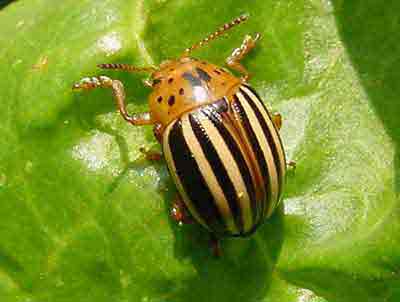This image captures a small, distinctive beetle perched on a green leaf. The beetle's head is a vivid reddish-orange adorned with black spots, and it features two prominent antennae. Its body displays a series of striking black and yellow stripes, reminiscent of a ladybug but with stripes instead of polka dots. The beetle's front showcases two long, leg-like extensions, while additional legs are visible underneath its body. The photograph is rectangular, highlighting the beetle's unique coloration and intricate design against the vibrant green background of the plant leaf.